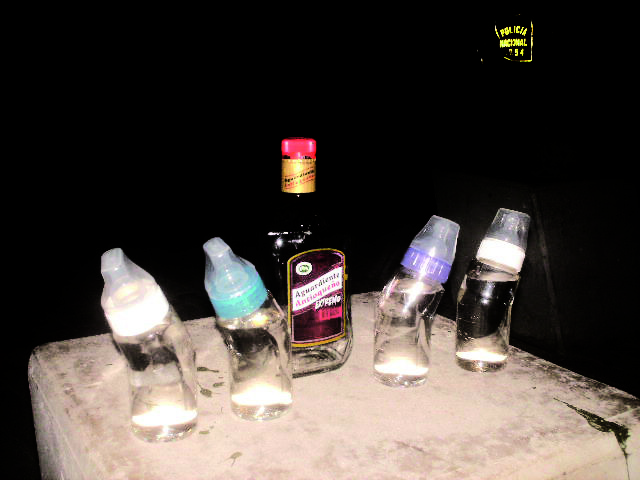In this image, a stark black background highlights a scene set atop a large ice block functioning as a table. Centered on this makeshift platform is a squat bottle of whiskey, distinguished by its red cap and gold label intricately detailed with black and red writing. Flanking this bottle symmetrically are four baby bottles—two on the left and two on the right. The baby bottles, filled with clear liquid that appears to be water, are designed with a slight bend for easier handling by infants. Each bottle features a plastic nipple covered by a screw-on cap, with two caps being white, one blue, and one purple. The detailed backdrop includes a dimly lit yellow sign, further enhancing the intriguing and unconventional composition of the photograph.